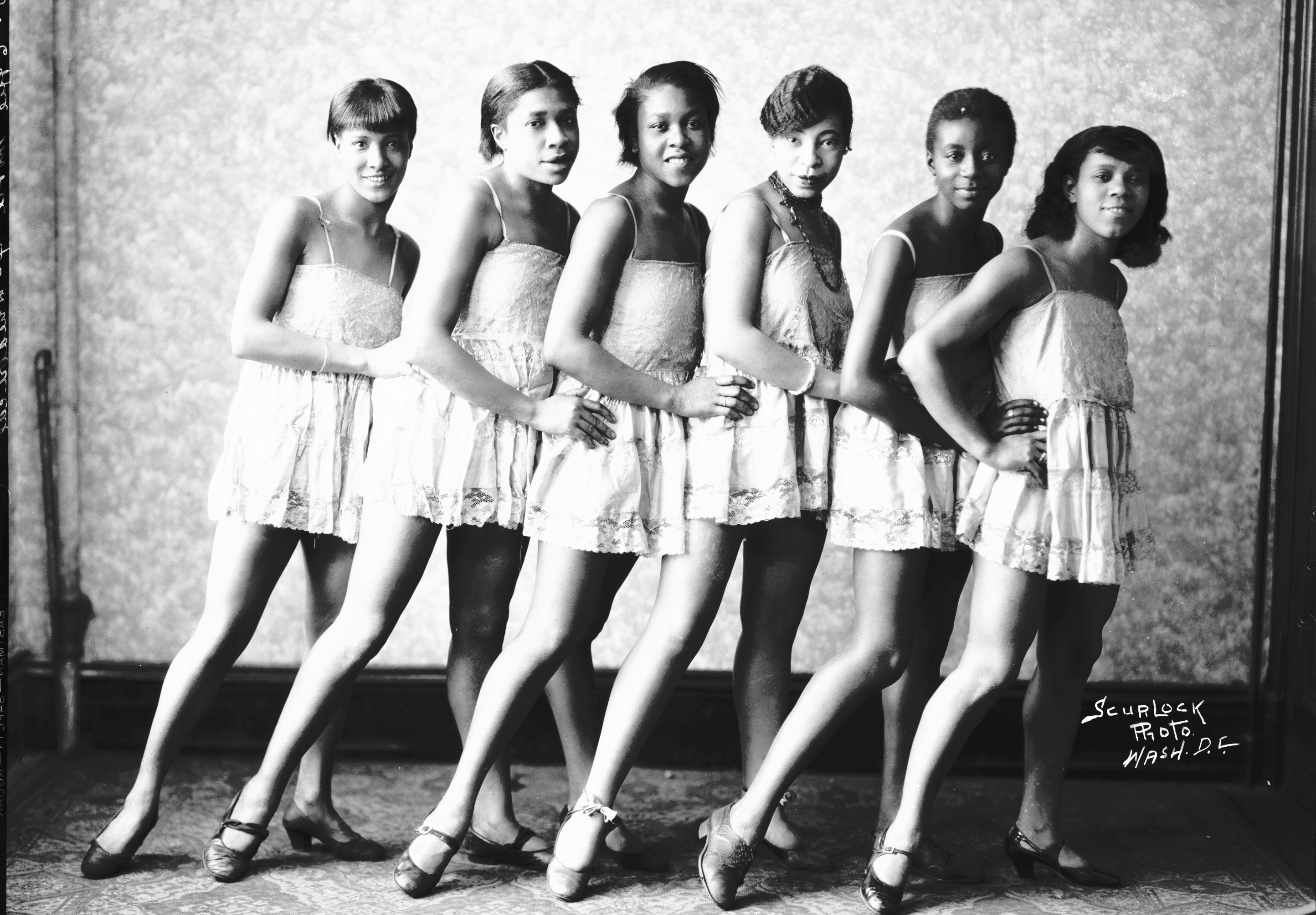This is a detailed black and white photograph, rectangular in shape, measuring approximately six inches wide and four inches high. The image captures six young African American women, standing in a lineup and slightly leaning to their right. They are positioned against a light-colored wall adorned with floral wallpaper and wood framing. The wallpaper features a pattern of blotchy tones in dark and light gray, while a dark, patterned carpet lies beneath their feet.

Each woman is dressed identically in short, thin-strapped dresses with a square neckline, which end just above the mid-thigh, revealing that the attire is quite risqué for the apparent time period. Their footwear consists of round-toed shoes, seemingly designed for dancing, suggesting that their outfits are dance costumes. In their pose, the women have their hands placed at each other's waists, except for the woman at the front who holds her own waist. Their hairstyles mostly feature short cuts, with the exception of the woman on the far right, who has shoulder-length hair.

In the bottom right corner of the photograph, there is white text reading "Scurlock Photo, Wash, D.C.," indicating that the photograph was taken by the Scurlock studio in Washington, D.C. This studio marking adds a historical and geographical context to the charming yet evocative snapshot of these young women.